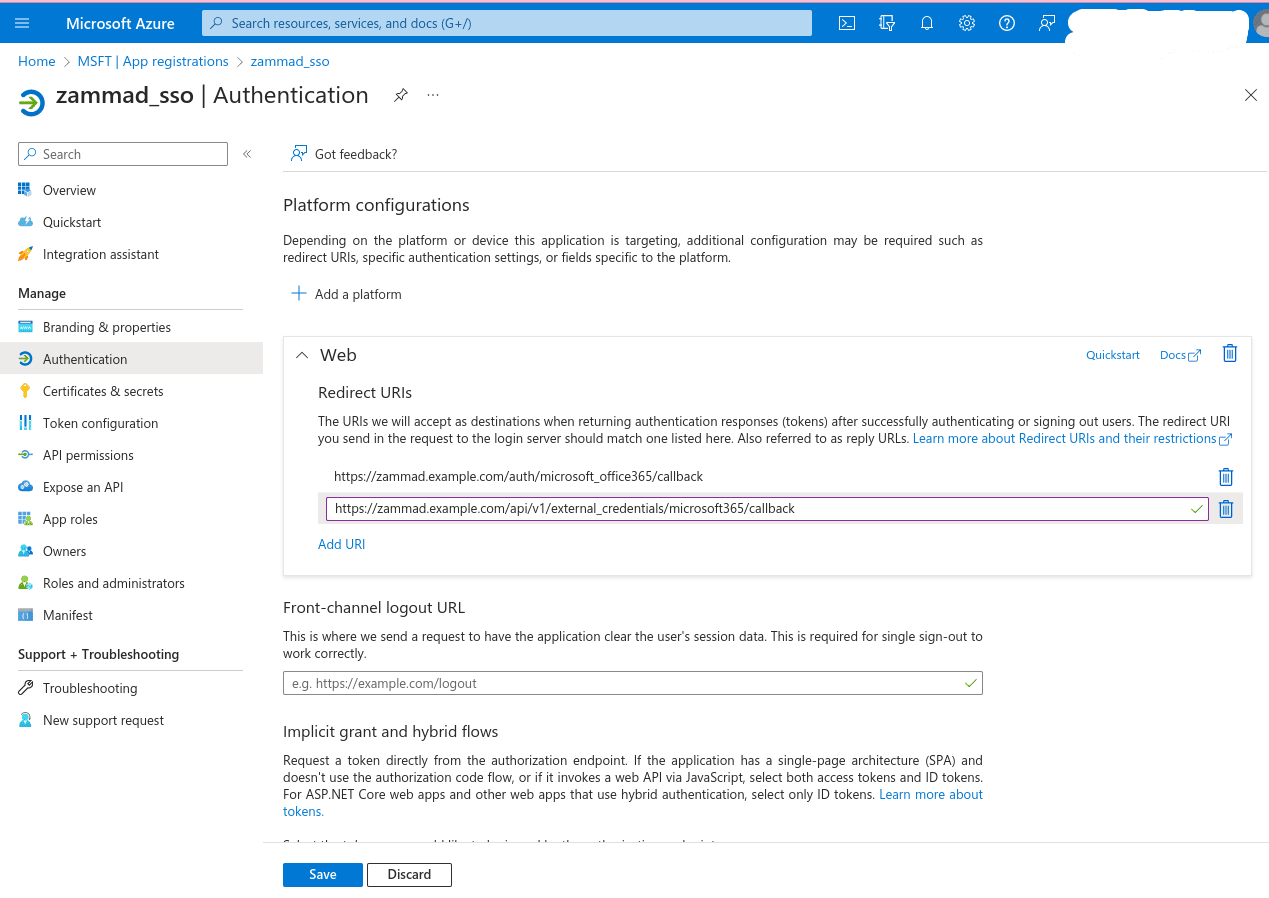This image displays the Microsoft Azure application, specifically highlighting the Zomed_SSO authentication settings. It illustrates a section dedicated to "Platform Configurations," which are essential for tailoring the application to specific platforms or devices. This configuration may involve setting up redirect URLs, fine-tuning authentication settings, or adjusting platform-specific fields. For instance, if a website needs to redirect traffic from an outdated link to a new site, the old URL and the new destination URL can be entered here to ensure a smooth transition. The authenticator app within Microsoft Azure helps secure these URLs, preventing them from redirecting users to potentially harmful websites. Overall, this feature within Microsoft Azure—an advanced cloud computing service—enhances web security and management capabilities.